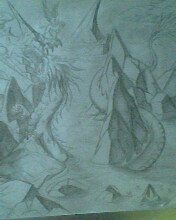The image is a detailed pencil drawing on white paper, featuring a heavily shaded, fantastical scene. Dominating the left side is a dragon-like creature with long frills or feathers sprouting from its head. Its tail curves in an intricate S-shape from the left to the right side, winding around a landscape of jagged rocks and sharp mountains. In the foreground, these rocks are particularly prominent, casting deep, heavy shadows. The background showcases a single, distinct triangular mountain, its peak slightly bent toward the upper right. The creature's scales and wing-like appendages hint at a hybrid nature, blending characteristics of dragons and serpents. The dark etchings contribute to a moody, almost surreal atmosphere, and the photo itself, though small and dimly lit, reveals a meticulously crafted, ribbon-like pattern that enhances the fantasy element of the scene. The ground appears to host water with objects seemingly floating, adding layers of depth and mystery to the composition.